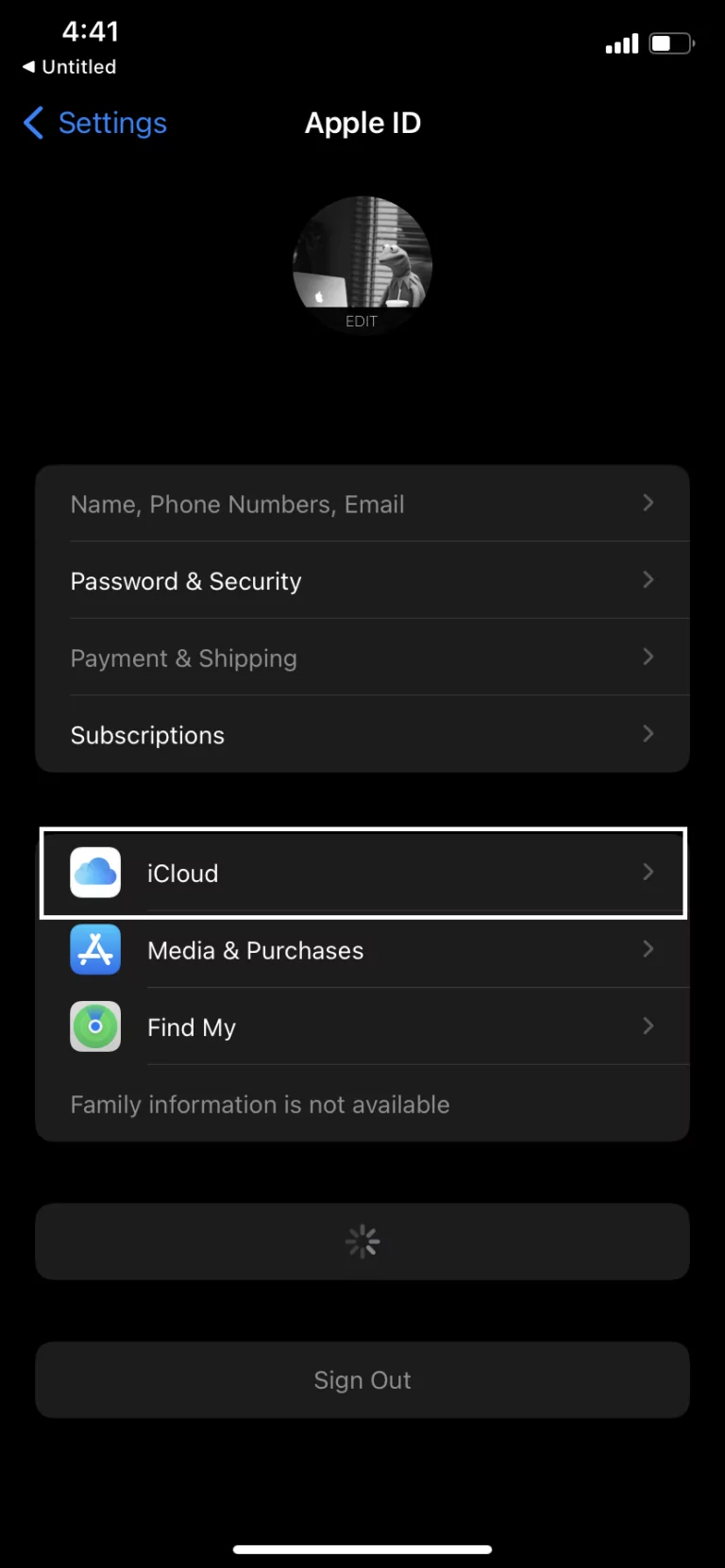A detailed screen capture of a smartphone shows a mostly black interface. At the top, the time is displayed as 4:41, followed by the label "Untitled" with a left arrow icon beneath it. The top right corner displays four signal bars and a battery meter at approximately 50%.

The main content begins with "Apple ID" and a circular profile image of Kermit the Frog inside a conference room, depicted sitting at a table with an open MacBook Pro in front of him. A window with louvered shades is visible in the background, along with a cup resembling those from McDonald's, partially in view at the top of the circle. Below the circular image is an "Edit" button, allowing changes to the profile image.

The interface continues with four major options on a gray background: "Name, Phone Numbers, Email," "Password & Security," "Payment & Shipping," and "Subscriptions." The "iCloud" option is currently selected, highlighted with a white rectangle around it. Additionally, "Media & Purchases" is listed next, featuring an 'A' logo on a blue field. Following that, a green icon resembling a radar map is labeled "Find My."

Further down, the screen shows the message "Family information not available" beside a loading icon within a gray rectangle, and beneath that, a red "Sign Out" button is prominently displayed.